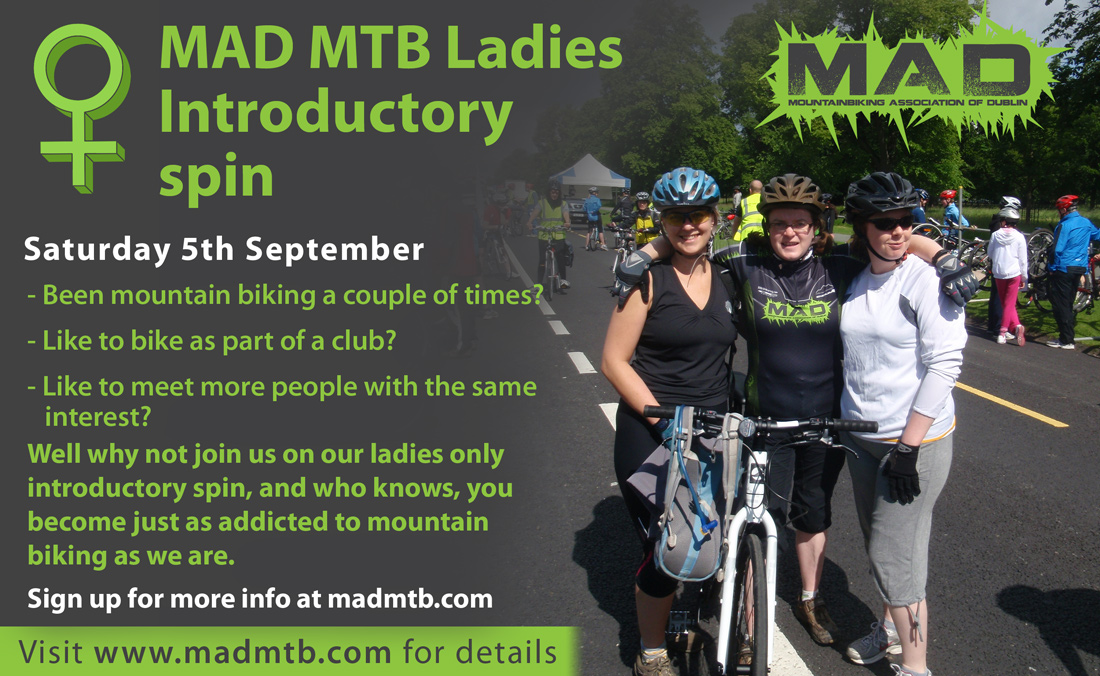The poster is predominantly grey on the left side, featuring a green symbol at the top left: a circle with a plus sign below it. Positioned at the top right corner, "MAD MTB Ladies Introductory Spin" is prominently printed in green. Beneath that, the date "Saturday, 5th September" is also in green. The detailed information includes three bullet points: "Been mountain biking a couple of times?", "Like to bike as part of a club?", and "Like to meet more people with the same interests?" Below these points, a paragraph encourages: "Well, why not join us on our ladies-only introductory spin? You might become just as addicted to mountain biking as we are." Additionally, the text "Sign up for more info at madmtb.com" is provided in white, followed by a green section on the right containing the word "MAD." At the bottom, there are three women wearing helmets, posing with their bicycles, illustrating the community spirit of the event.